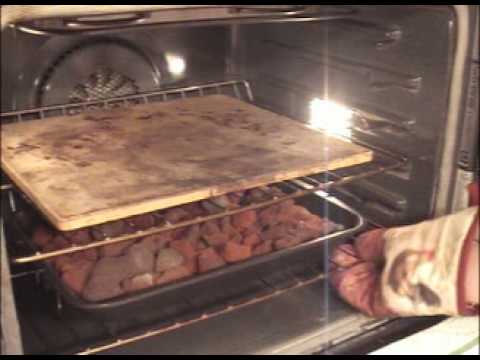The image depicts the interior of a gray, metallic oven with its light on, seen from an outside angle that showcases the back and right side, but not the left. The oven contains two silver racks. On the upper rack lies a thin, flat surface which appears to be a stained stone or wooden cutting board with marks from various foods. The lower rack holds a sizable black pan that spans the oven's width, containing small pieces of meat, possibly chicken. A hand, adorned with a red and white oven mitt featuring a rooster design, reaches in from the right to grasp the bottom rack. The photo is slightly blurry, lending it a vintage feel reminiscent of the 1970s or 1980s.